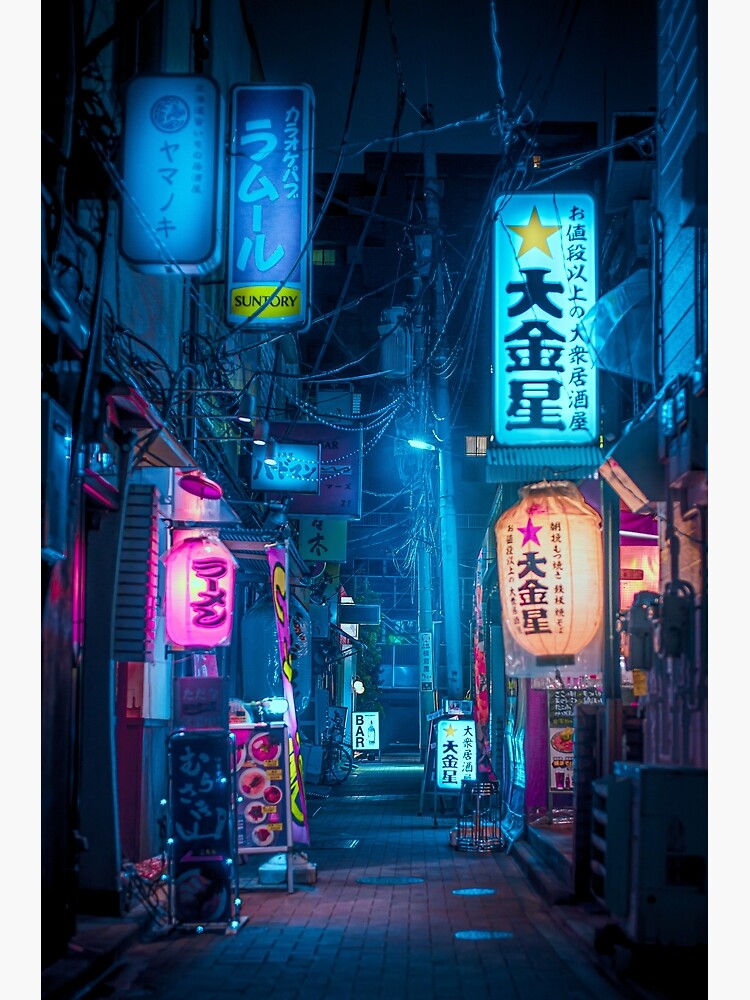The image depicts a narrow, brick-paved alleyway in a city at night, likely in Japan or China, given the prevalence of foreign characters resembling Japanese or Chinese script. The alley is flanked by numerous stores, adorned with vibrant neon signs in hues of blue, pink, and orange. On the left side, two blue-lit signs hang from a building, one of which vertically spells out a word ending in "sundry" in yellow. At the base of this building, pink neon signs cast a colorful glow. Wires dangle in front of the structure, adding to the intricate urban detail. The right side showcases additional buildings with a yellow star-adorned sign bearing vertical foreign letters and a glowing paper lantern featuring a pink star and similar script. The scene is devoid of people, evoking a serene, almost cinematic atmosphere perfect for a night-time stroll, akin to settings often seen in movies or manga.